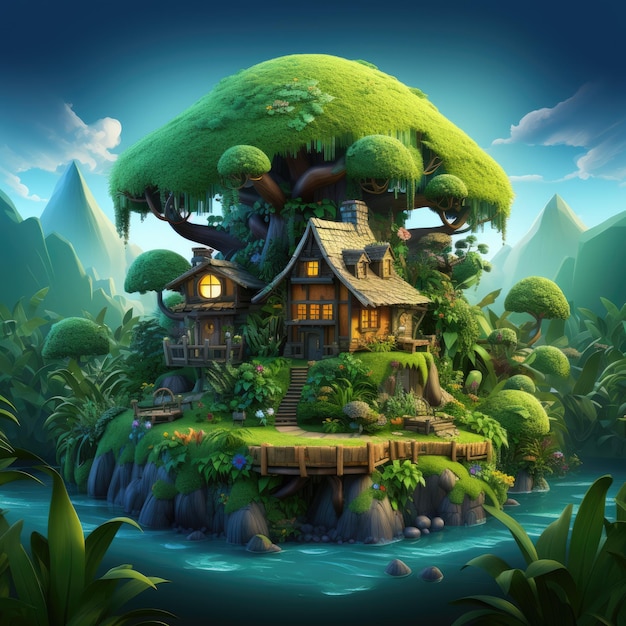The image is a detailed 3D digital drawing in a cartoonish, Pixar-style animation, depicting an idyllic scene centered around a tree house. Perched atop a rocky island surrounded by water, the setting includes a main cottage-style house and a smaller adjacent house situated beneath a sprawling tree with a canopy resembling a mushroom. The scene is lush with greenery, featuring grass, flowers, and mushroom-shaped trees. A set of stairs leads up the hill to the tree houses, with the illuminated windows casting a warm glow. In the background, a range of mountains frames the clear blue sky, dotted with white clouds, creating a picturesque setting that might belong in a children's book or movie.